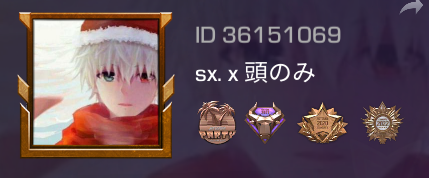The image is a small, indigo or navy blue rectangle with an anime-style theme, likely a screenshot from a game or app. Dominating the left half is an ornate, gold-framed illustration of a character with distinct features. The character has white, spiky hair, a serious expression, heterochromatic eyes with the right eye being red and the left green, and is dressed in a red outfit, either a hat with a white trim resembling a Santa hat or a dark red sweater. The background within the frame includes a snowy scene. 

To the right of the framed character, there is white text displaying "ID 36151069" and beneath that, another line of text that reads "SX.X" followed by some Asian characters. Below the text, there are four emblems or medals, predominantly gold and brown, with touches of rust, purple, and blue. Additionally, at the top right corner of the image, there's a small arrow pointing to the right.